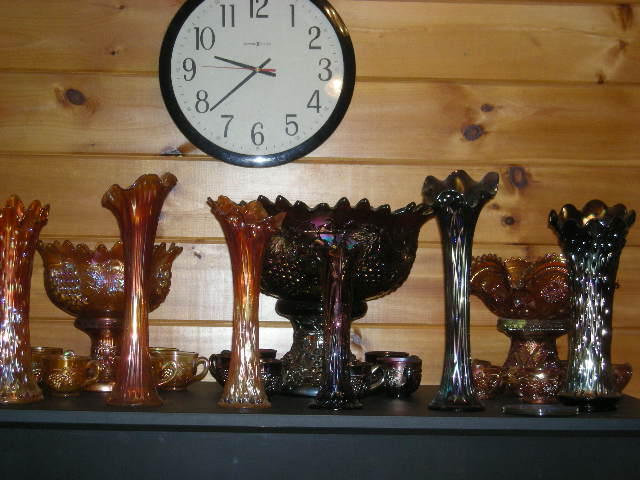The image captures a detailed snapshot of a mantelpiece adorned with an ornate collection of glassware. The scene features a background of pale wooden paneling with visible knot holes, suggesting a rec room environment. Central to the composition is a black plastic analog clock on the wall, displaying the time at 9:38, with its top slightly cropped in the frame.

The mantelpiece itself, crafted from black wood, supports an array of intricately designed glass items. These include tall, fluted vases and shallow bowls, all characteristic of carnival glass. Their colors range from iridescent golden amber to dark shades of obsidian, onyx, and purple, with some pieces having an opalescent quality. The vases vary in shape, with some resembling pitcher plants—long and slender with wide tops. Others are more bowl-like, sitting on glass bases, accompanied by glass teacups in similarly diverse hues.

One particularly notable design feature on the darker glass items is a detailed grape motif, adding to their ornamental charm. This carefully arranged display on what appears to be a tall dresser or shelf in front of the clock creates a visually captivating and richly textured centerpiece for the room.